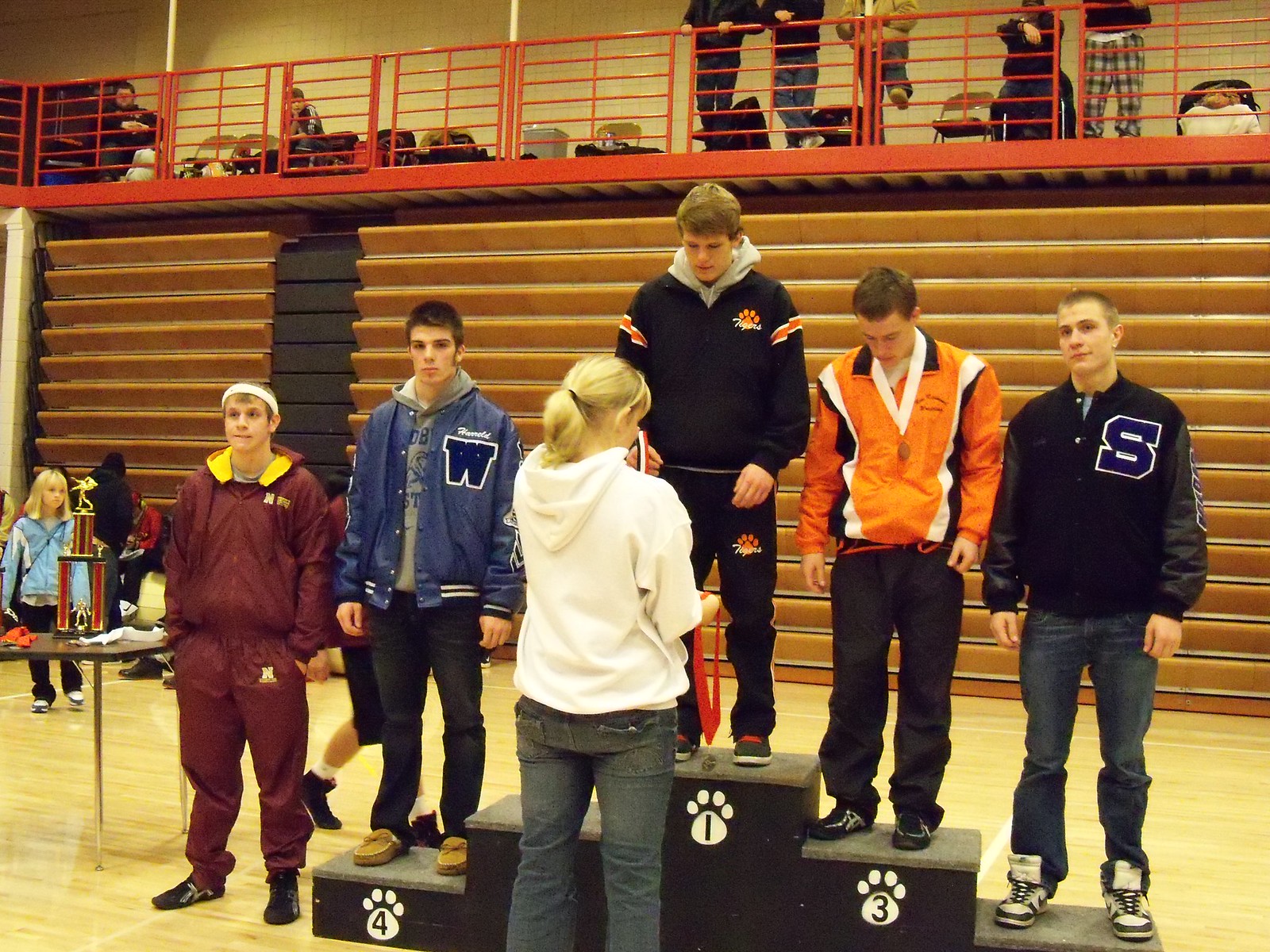A detailed photograph of an indoor award ceremony, likely held in a high school gymnasium, features a multi-level black wooden podium with five levels marked by white paw prints. The first, third, fourth, and fifth positions on the podium each have a young man standing on them, while the second-place spot is curiously empty. Another young man stands on the floor to the left of the podium. All the participants appear to be high school boys wearing different colored varsity jackets, indicating they might be from different schools. The young man in the third-place position has already received a medal, and a woman with blonde hair, dressed in a white hoodie and blue jeans, is in the process of awarding a medal to the first-place winner. A table to the left of the scene holds a trophy. Behind the podium, the gym bleachers are folded up against the wall, while a few spectators can be seen in the background, looking on from an elevated area above the stands. The gym’s glossy wooden floor adds a polished feel to the overall setting.